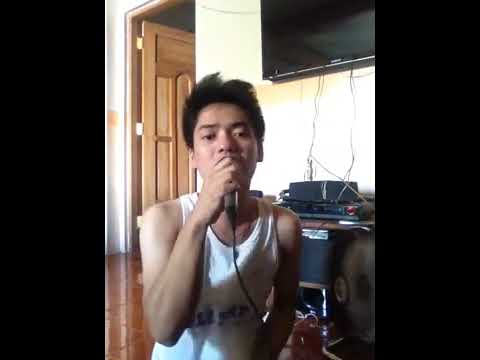The image depicts a young Asian boy with short black hair, styled upwards. He is wearing a white tank top and is positioned in the middle of a living room, visible from the waist up. The boy is either standing or sitting on the ground, directly facing the camera, and is holding a black, corded microphone close to his mouth with his right hand, appearing to be singing or speaking.

The room itself features off-white walls and a polished hardwood or reddish clay tile floor. Behind the boy, on the right-hand side, there is an open doorway with a light brown wooden door. Adjacent to this is a wall-mounted black TV with several messy cables hanging down, connecting to a crude entertainment center or dark brown wooden shelves below. Various components, such as a black speaker bar and other electronics, are placed on these shelves, contributing to the somewhat cluttered appearance.